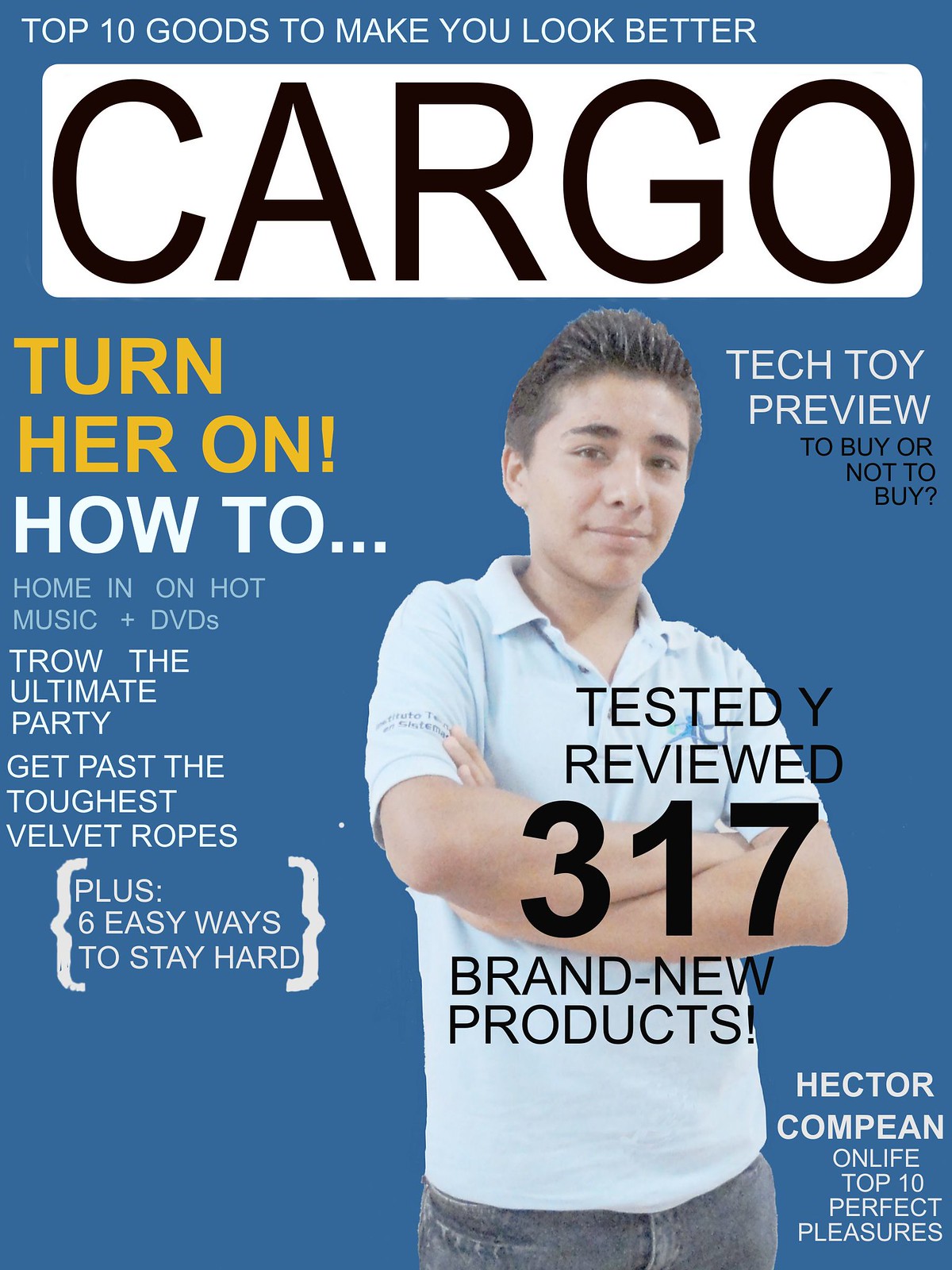The image features a detailed magazine cover mock-up with a solid blue background. At the very top, there is white text that reads "Top 10 Goods to Make You Look Better." Below that, a white rectangle with large black capital letters spells out "Cargo." Along the left margin in yellow text, it says "Turn Her On." Following that, in white text, the cover reads "How To: Home In on Hot Music Plus DVDs, Throw the Ultimate Party, Get Past the Toughest Velvet Ropes, Plus 6 Easy Ways to Stay Hard." On the top right margin, black text reads "Tech Toy Review: To Buy or Not to Buy. Tested, Reviewed, 317 Brand New Products." 

On the right side of the cover, there is an image of a young man, likely in his teens or early 20s, with a white complexion. He is wearing a white short-sleeved polo shirt and gray jeans, posing with his arms crossed. Overlapping the image, black text reads "Tested, Reviewed, 317 Brand New Products." To the right of the image, it says "Tech Toy Review: To Buy or Not to Buy." In the bottom right corner, it reads, "Hector Compeán on Life: Top 10 Perfect Pleasures."